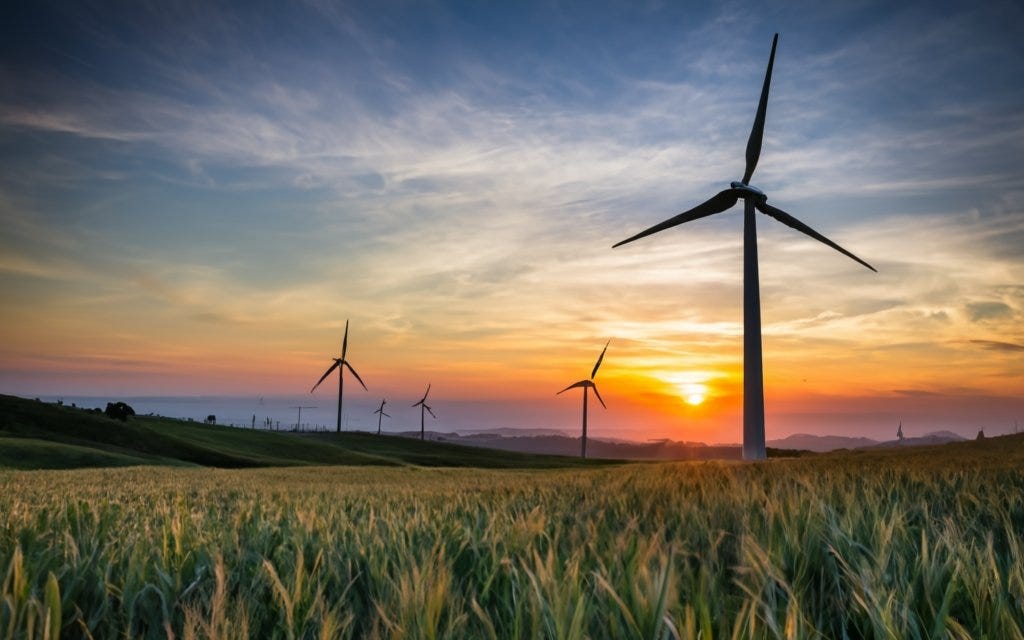The image depicts a serene landscape at sunrise featuring a wind farm with five wind turbines prominently arranged across a field. The sun, with its bright yellow light, hovers near the horizon between two central windmills, creating a striking contrast against the colorful sky. The upper part of the sky retains a deep blue hue, transitioning into shades of yellowish-orange and purple closer to the ground. White clouds linger near the horizon, contributing to the tranquil atmosphere. In the foreground, tall green and yellow grasses stretch across a third of the image, giving way to what appears to be a body of water in the mid-ground, hinting at a touch of blue. To the left, a low mountain slope adds dimension to the landscape. The windmills, evenly spaced from the foreground to the horizon, stand tall over the rolling hills, emphasizing the expanse and peacefulness of the scene.